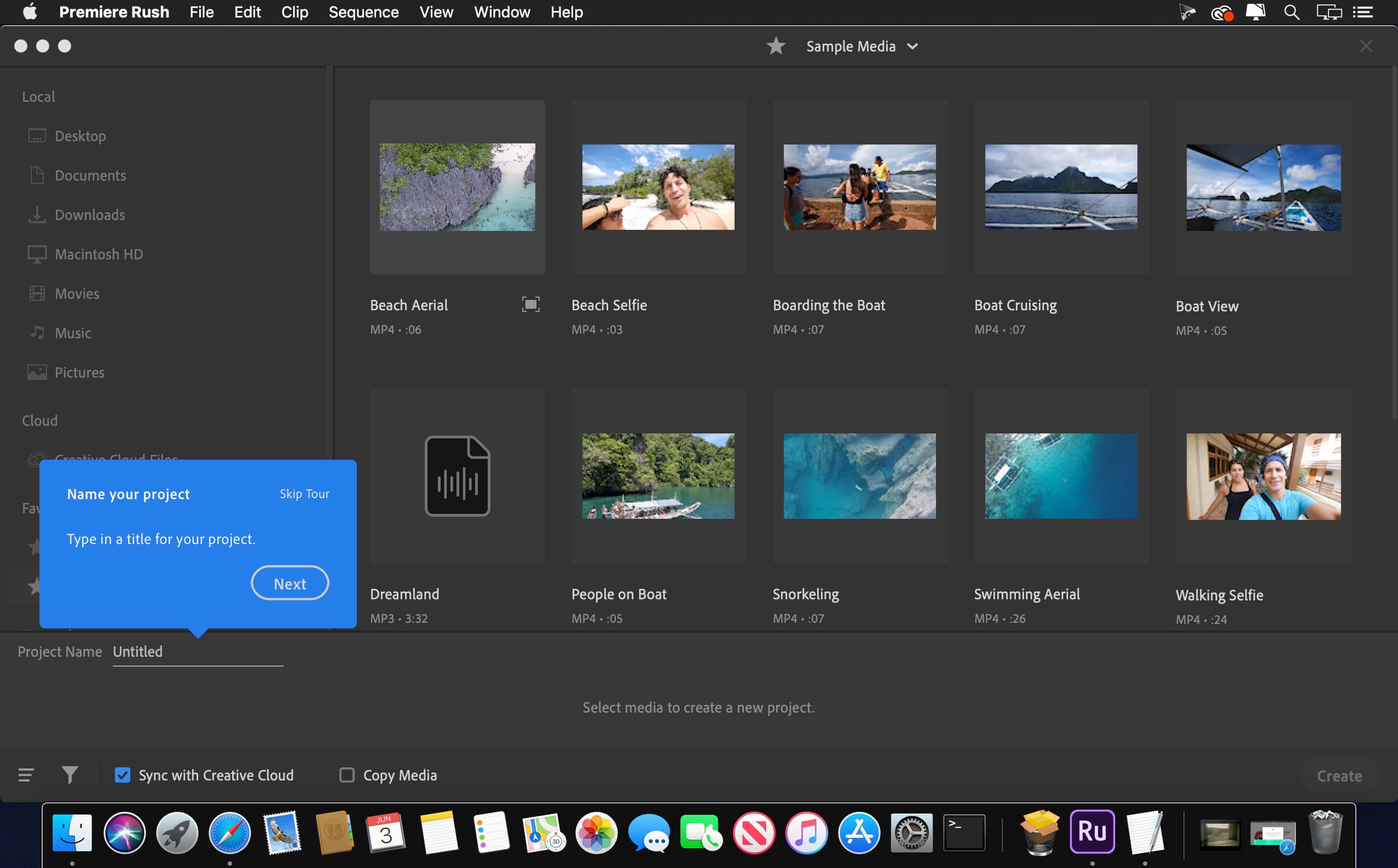Screenshot showcasing the Premiere Rush video editing app on an Apple device. The app's interface displays a webpage with various sample media files in MP4 format that users can experiment with. The main section prominently features these samples, ready for editing. At the bottom of the screen, there's a prompt for naming the user's project, currently labeled "Untitled." A blue checkmark indicates that syncing with Creative Cloud is enabled, although the media files have not been copied yet. On the left side of the screen, several navigation options are visible, including local desktop, documents, downloads, Macintosh HD, movies, music, and pictures, providing multiple sources from which users can import files.